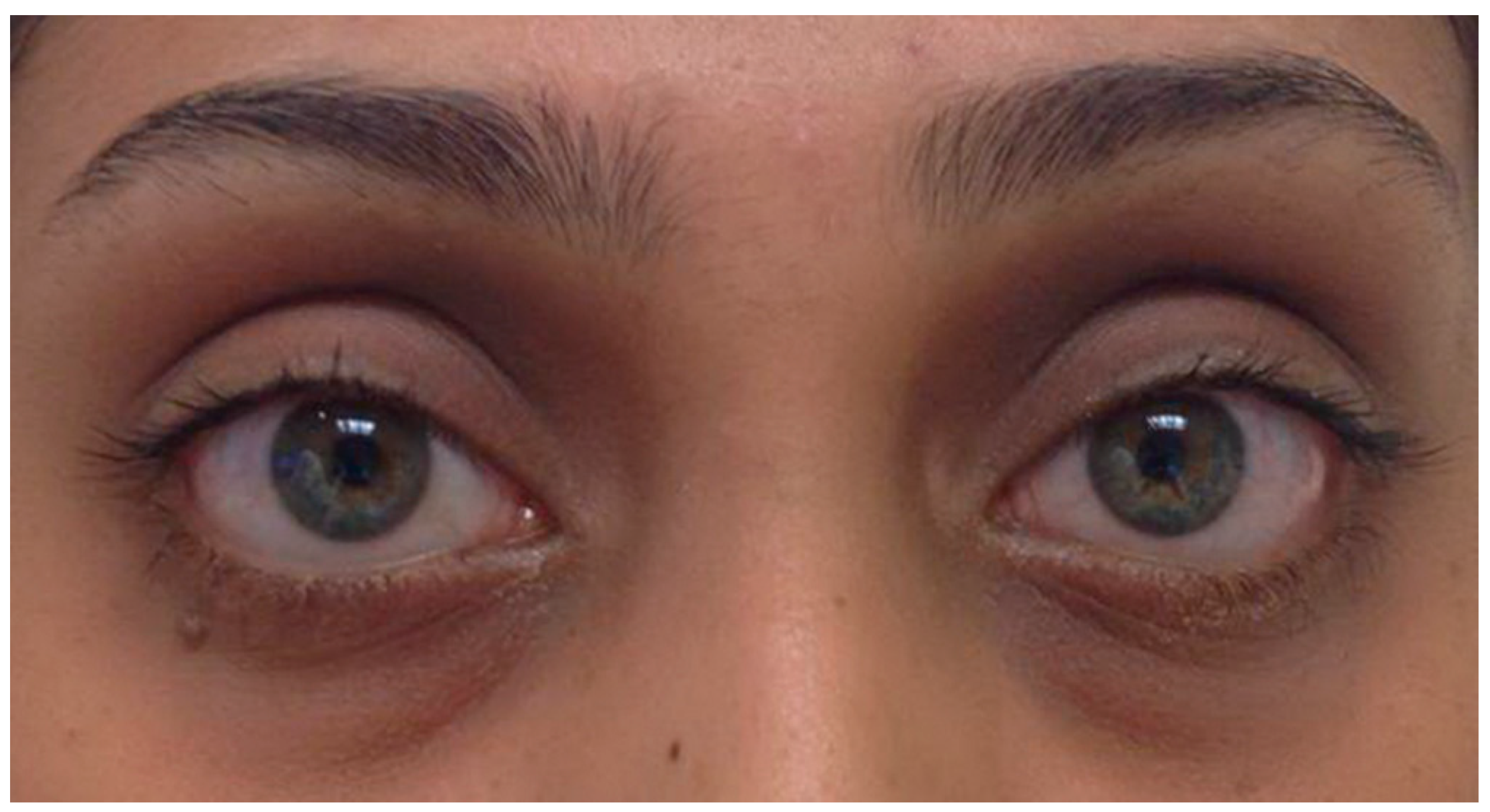This extreme close-up image showcases the central T-zone of a woman's face, highlighting her hazel green eyes, which blend hints of bluish-green on the outer edges and a touch of brown nearer to the pupils. Her complexion is light brown, and her messy yet curvaceous dark brown eyebrows frame her eyes. A small mole is visible underneath her right eye, alongside a noticeable brown freckle on the lower side of her nose and another smaller freckle on the upper left side of her nose bridge. Her eyelashes appear clumped, possibly due to makeup, adding to the tired look underscored by subtle dark circles and slightly pink, dry eyes. Despite a fair complexion, areas like the mole and freckles add uniqueness to her facial features.